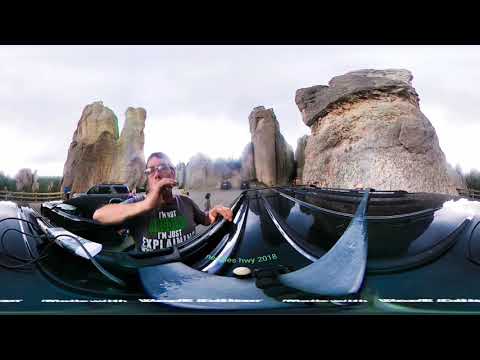In this 360-degree fisheye image, a man, wearing glasses and a dark gray t-shirt with the partially visible text "I'm just explaining," is standing next to a vehicle. He holds a selfie stick in his left hand, raising his right forearm to his mouth in a semicircle shape. The t-shirt details include white and green text. The scene around him features the roof of a vehicle with shiny, metallic components, possibly a car, a van, or even a boat. Behind him, the landscape reveals striking rock formations that tower upward, suggesting a national park setting. The background is populated with various SUVs and vans, and there are some pedestrians near a wooden fence. Over the scene, a white, cloudy sky looms, adding to the natural ambiance. The image also contains watermarks with the text "Highway, HWY, 2018," hinting at the location or context.